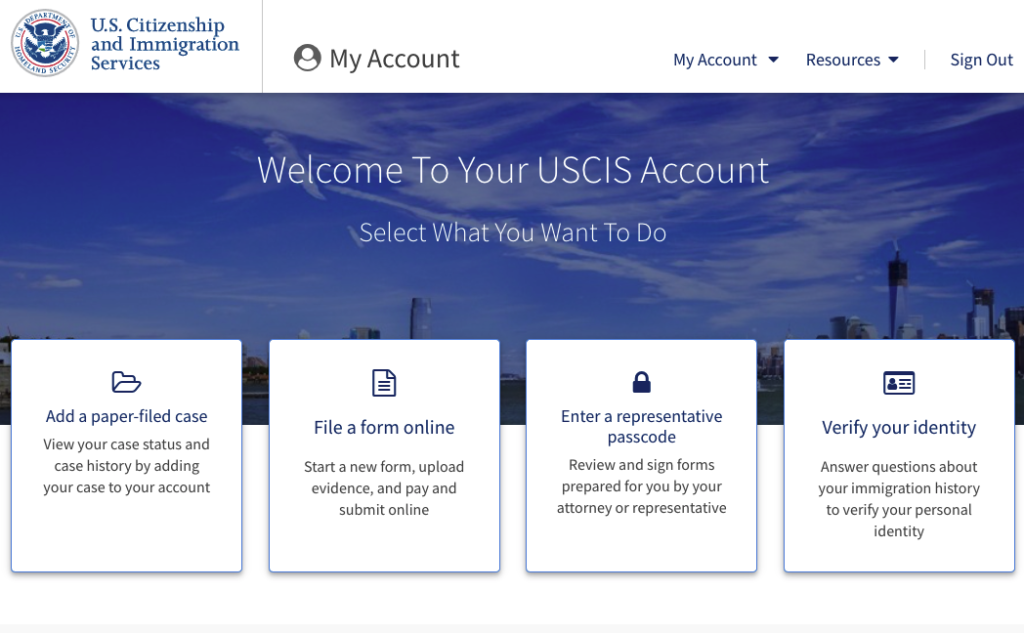This image is a screenshot from the U.S. Citizenship and Immigration Services (USCIS) website, captured on a computer. Positioned at the very top left corner, the image displays the text "U.S. Citizenship and Immigration Services" on a white background, accompanied by the USCIS seal. To the right, a gray section shows "My Account" along with a default account logo icon. Further to the right, dropdown menus labeled "My Account" and "Resources" are displayed in blue text, followed by a "Sign Out" option.

Below this top navigation bar is a scenic image of the sky, featuring a faint city skyline in the background. Overlaying the sky image is white text that reads, "Welcome to your USCIS account." In smaller text just beneath, it states, "Select what you want to do."

The central section of the image consists of four white squares, each bordered by a thin, light blue line and slightly overlapping the white background. Each square contains an icon and descriptive text:
1. The first square has a file icon and reads, "Add a paper-filed case." It also mentions, "View your case status and case history by adding your case to your account."
2. The second square features an icon of a piece of paper and says, "File a form online." It details, "Start a new form, upload evidence, and pay and submit online."
3. The third square displays a lock icon and instructs, "Enter a representative passcode." The accompanying text explains, "Review and sign forms prepared for you by your attorney or representative."
4. The final square shows an ID icon and states, "Verify your identity." The additional text specifies, "Answer questions about your immigration history to verify your personal identity."

The rest of the screenshot maintains a clean and simple white background, emphasizing the structured and user-friendly layout of the USCIS portal.